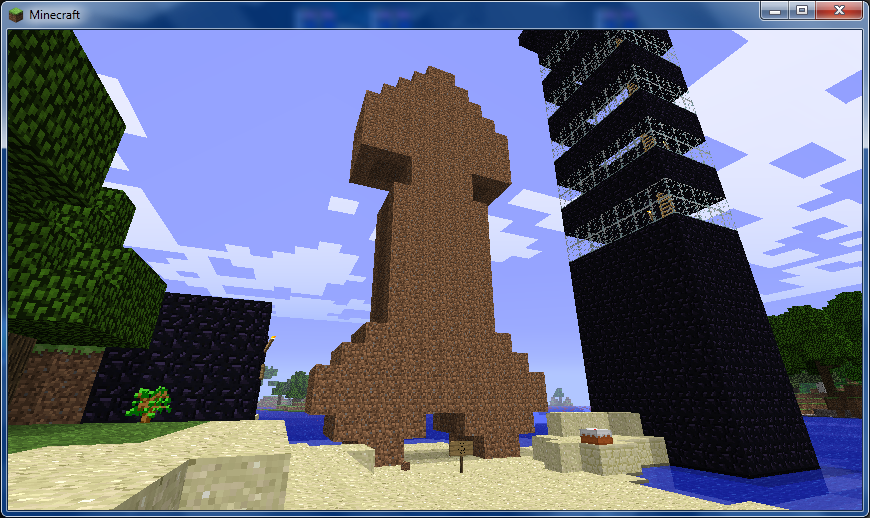The image is a highly pixelated screenshot from the video game Minecraft, as indicated by the game title in the upper left corner along with the window control buttons. The scene features a light beige-gray paved plaza area at the bottom center. On the left side of the image, there's a dark brick wall and a green tree with square-shaped leaves, rooted in dark brown dirt. Beside it is a green plant emerging from a black square. In the middle of the plaza, a large, brown arrow-like structure stands prominently, resembling a statue. To the right, a blue water body is depicted with a vivid, bright blue shade that contrasts with a tall, black-and-clear windowed rectangular tower rising from it. The tower consists of alternating black strips and clear windows. Behind the tower, green trees with brown trunks are visible. The sky above is light purple with large, white, geometrically squared clouds. Overall, the image combines various elements typical of the Minecraft style, displaying a mix of natural and architectural features in a pixelated, colorful composition.